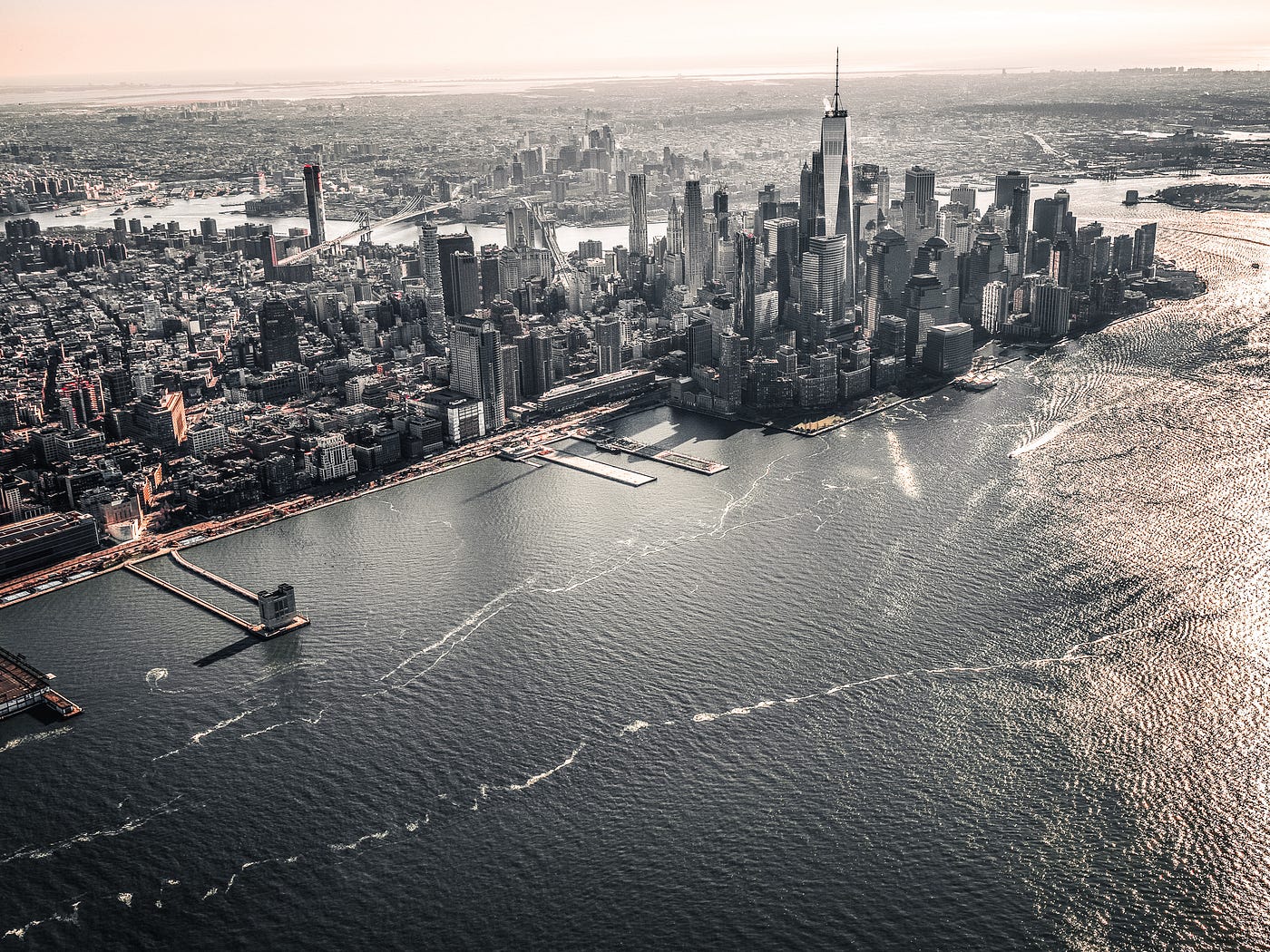This black and white aerial photograph captures an extensive view of what appears to be New York City, taken just as the sun is about to set. The camera is elevated about 100 feet above the ground and positioned over a large body of water, most likely a bay, looking slightly to the right. The foreground features the calm, sunlit waters with visible ripples and white streaks hinting at boat activity. Stretching from the left to the right edge of the image, the shoreline reveals ports and piers jutting into the water. Dominating the city's skyline are numerous tall skyscrapers, high-rise buildings, and a dense cluster of various residential and commercial structures. In the background, the sprawling metropolitan area extends further, showcasing a vast urban landscape. On the left side of the image, a bridge spans the water, connecting different parts of the city. The sky, visible in the top one-tenth of the photograph, adds to the dramatic ambiance as daylight fades.